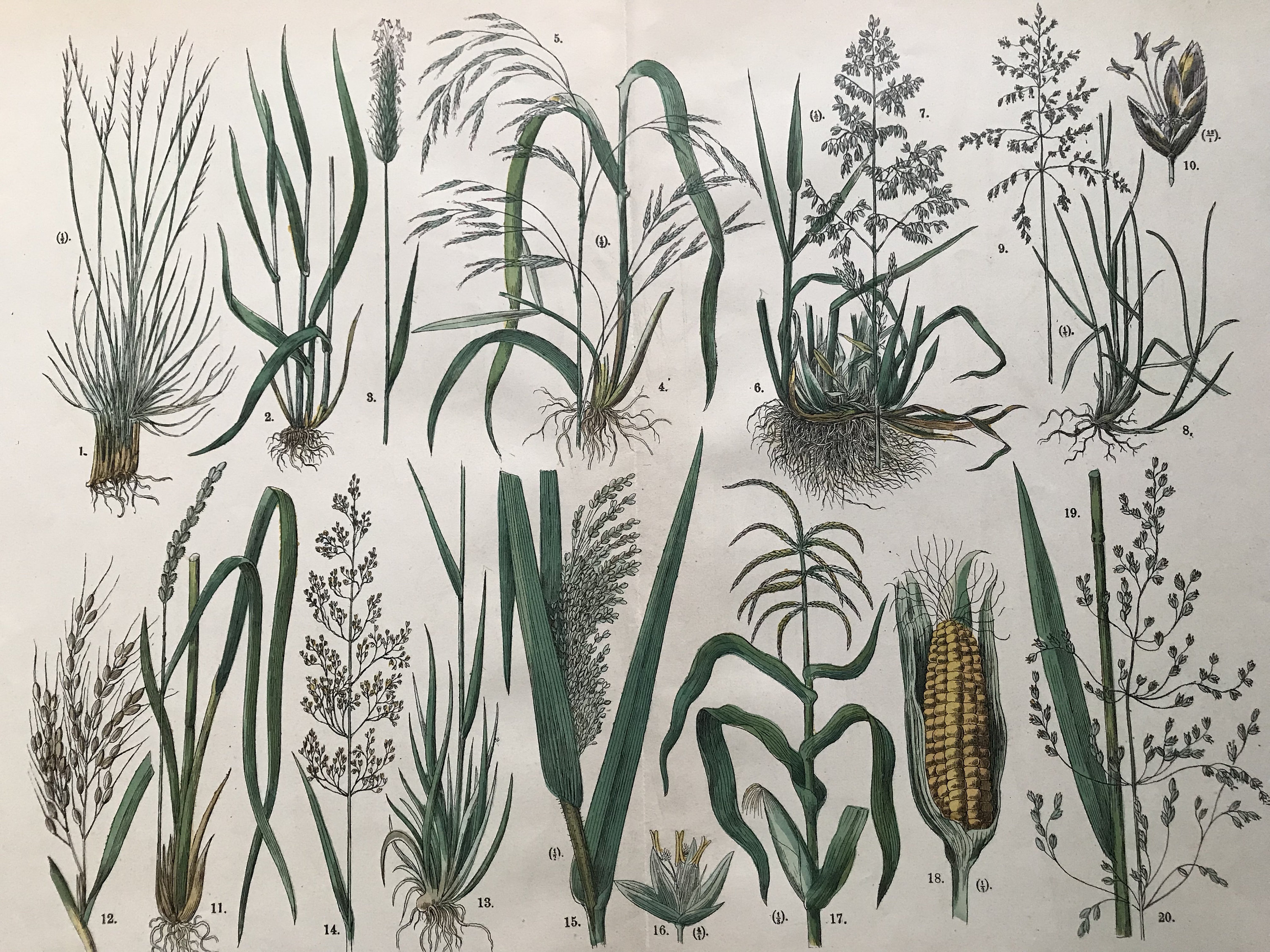This detailed illustration appears to be a historical botanical plate, likely from an old book or magazine, depicting various plant specimens with a focus on cereals and grasses. The image is organized in two rows, each showcasing multiple plant species, which are labeled with numbers ranging from 1 to 20. These plants are predominantly characterized by their long stems and grassy appearances. 

On the far left, a plant with tall, thin grasses that fan out at the top with tiny spikes is noticeable. Adjacent to it, there is a specimen with broader leaves and longer stems. Another plant features a long stem with a flowery, grain-like top, akin to a cattail but not quite the same. Next to it, there is a plant resembling wheat with thin protrusions and grain-like structures that bend over slightly from the weight. Further along, there is a stalk with tree-like branches and various leaves at the top, suggestive of another grain.

The most distinct features on the bottom row include an ear of corn prominently displayed on the bottom right (number 18) and a nearby corn stalk with thick leaves and a flowering top (number 17). The numbered illustrations, likely representing different stages of plant growth or different types of cultivated crops, convey a broad spectrum of plant morphology. The visual differences among them include variations in stem thickness, leaf structure, and flower or grain presentation, suggesting a diverse collection of cereal plants and grasses. This intricate and methodical presentation offers a glimpse into historical agricultural study and botanical illustration.